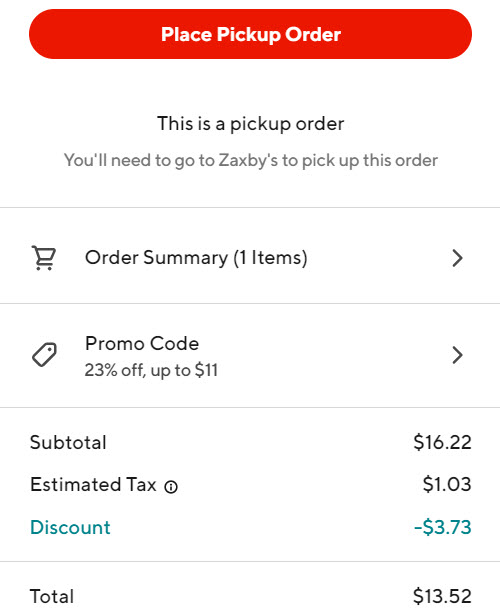Screenshot showing an order summary for a Zaxby's pickup. At the very top, there is a prominent red box with white text reading "Place Pickup Order." Below it, in black text, is a message stating, "This is a pickup order." In lighter gray text, it instructs, "You'll need to go to Zaxby's to pick up this order," separated by a horizontal line for clarity.

A shopping cart icon is visible on the left, adjacent to the text "Order Summary" in black. Next to this, in parentheses, it's noted in black text that there are "1 item," followed by a small black arrow pointing to the right.

Following another separating line, there is a "Promo Code" section with black text and a small coupon icon to the left. It mentions "23% off up to $11" in lighter gray text, accompanied by another black arrow pointing right. 

Below this section, separated by a line, the subtotal is displayed in black text on the left with the amount "$16.22" on the right. Beneath the subtotal is "Estimated Tax" with a small upside-down exclamation mark inside a circle, indicating the amount "$1.03" on the right. Under this, a teal-colored text states "Discount," showing a deduction of "-$3.73" to the right.

The final line separates these details from the "Total" section, where the total amount of "$13.52" is displayed in black text on the right.